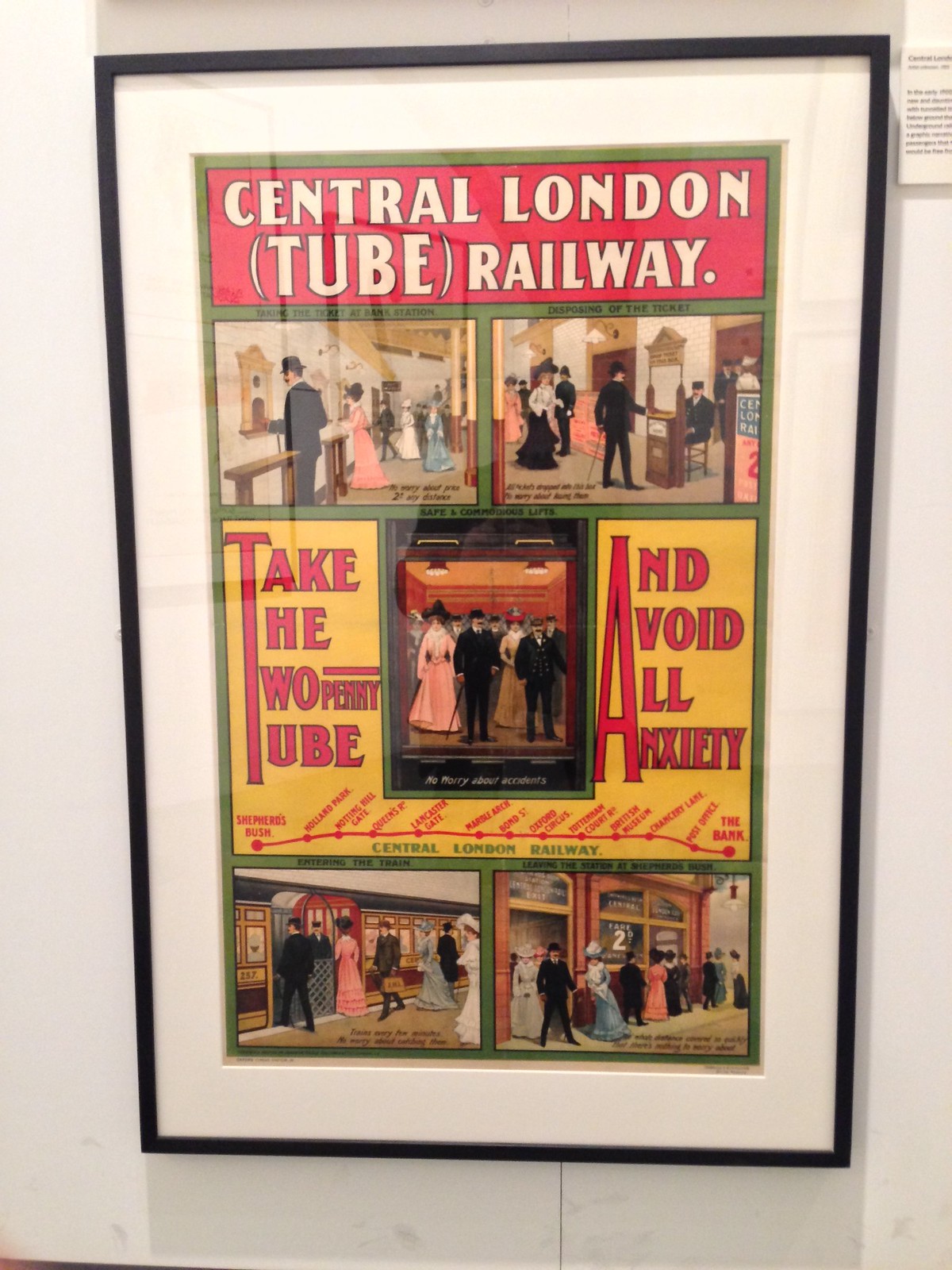In a framed vintage artwork, edged in a sage green hue and encased in a thin black frame with a white matting, an advertisement for the Central London (Tube) Railway captures the viewer's attention. The top of the artwork features a bold red box with the words "Central London (Tube) Railway" in striking white letters. Below, two illustrations depict historical scenes, likely from the early 20th century, showing individuals dressed in period attire such as suits, gowns, top hats, and canes, reminiscent of the 1920s-1940s era. Positioned strategically in red text, the slogan "Take the two penny tube and avoid all anxiety" connects past travelers' ease with modern-day convenience. A schematic representation of the railway line follows, marked with station names such as Shepherd's Bush, Holland Park, and Oxford Circus. At the bottom, additional illustrations portray passengers from the same bygone era, waiting at a train station, adding further depth to the historical ambiance. The entirety of the artwork is displayed against a white wall, potentially suggesting its placement in a museum or a gallery.